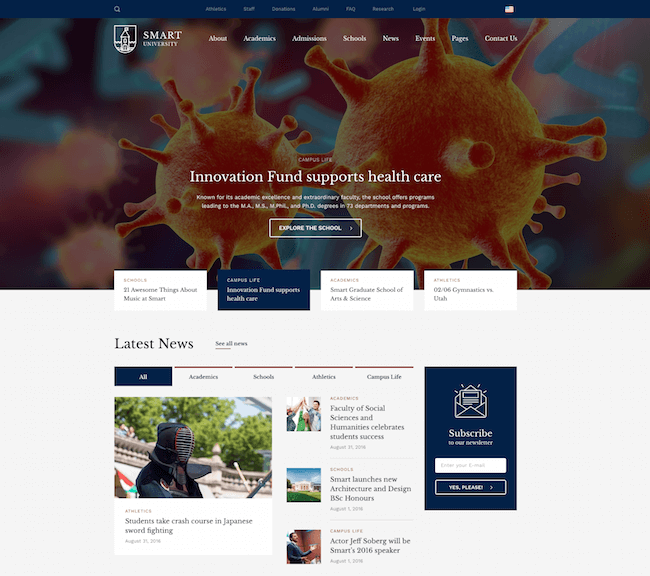The top of the image features a banner with a blue background and white text. At the center of this banner, the words "Smart University" are prominently displayed alongside a logo resembling a shield with a tower emblem. This blue band at the top includes several navigation links, though some are difficult to read. Identifiable links include FAQs, Research, and Login, with possible additional links for Donations/Donors and Staff.

Below this banner, aligned with the "Smart University" heading, are more navigation options: Academics, Admissions, Schools, News, Events, Pages, and Contact Us. On the far right of the blue banner is a small American flag icon.

The background image showcases a close-up of viruses, depicted as spherical structures with protruding spikes. Superimposed on the lower center of this image, there is white text reading "Innovation Fund Supporters Healthcare."

Beneath this, in white text, a statement celebrates the university: "Known for its academic excellence and extraordinary faculty, the school offers programs leading to the MA, MS, M[unknown]A, and PhD degrees in 73 departments and programs." Additionally, there is a button labeled "Explore the School."